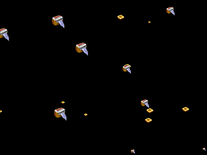This image, which appears small and possibly shrunken down, showcases an art piece or a scene resembling an old video game, set against a very dark black background. The rectangular image, wider than it is tall, depicts several objects that resemble spaceships or toasters with wings. These objects feature a range of colors, including silver, white, red, and hints of brown or orange, with prominent blue wing-like extensions. The spacecraft-like objects vary in size and are scattered randomly across the scene. Alongside these, there are yellow and orangish-yellow disks of different sizes, which might represent stars or other celestial bodies. Two white dots also appear, one at the bottom and another in the lower right-hand corner, adding to the intricate composition of the image. The overall impression of the image is reminiscent of a vintage video game, possibly like Space Invaders, where the objective might involve shooting at these various objects.